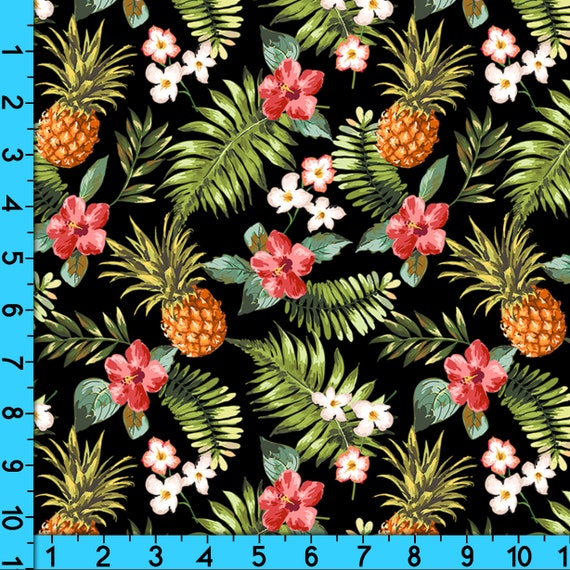The image features a square measuring device overlaid on a tropical-themed background. The device has blue rulers with black markings running along both the left edge and the bottom edge, numbered 1 through 10. The background is a vibrant, repeating pattern that includes various tropical flowers and pineapples. The flowers are predominantly red and pink, with some white flowers that have yellow centers and pink or pink-outlined petals. The lush foliage depicted includes large green leaves, shaded with hues of dark and light green, evoking the feel of a Hawaiian shirt print. Overall, the scene combines precise measurement tools with a lively and colorful tropical design.